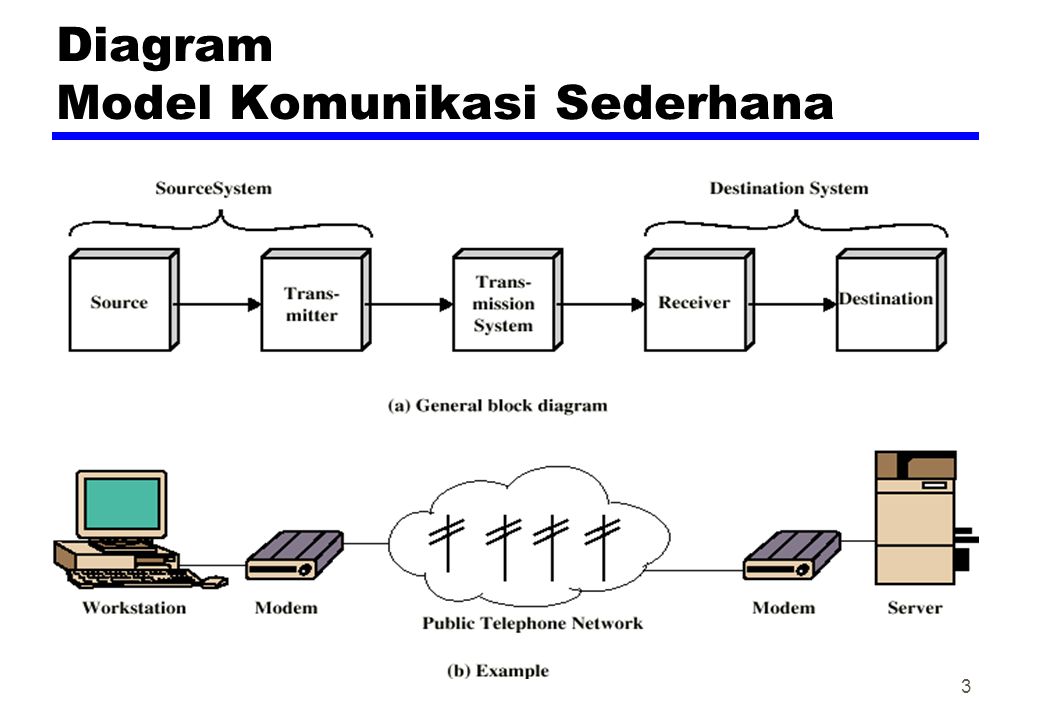This image is a detailed digital diagram with a central theme of communication. The layout is set against a white background, with the title "Diagram Model Komunikasi Sederhana" prominently displayed in bold black letters at the top. Directly beneath the title, a blue horizontal line extends from left to right. The main focus of the diagram is a sequence of five small boxes arranged horizontally in the center, each connected by right-pointing arrows. These boxes are labeled in the following order: "Source," "Transmitter," "Transmission System," "Receiver," and "Destination." The "Source" and "Transmitter" boxes are grouped together under a label "Source System," while the "Receiver" and "Destination" boxes are grouped under a "Destination System" label.

Below the primary diagram, there is a secondary illustrative sequence depicting an old-style computer labeled "Workstation," which connects to a "Modem." This modem is linked to a cloud icon symbolizing the "Public Telephone Network," featuring telephone line symbols. The sequence continues with another modem leading to a depiction of an old server labeled "Server." The visual elements of the diagram are accentuated with colors such as black, white, blue, green, tan, gray, and various shades of brown, giving it a retro and utilitarian appearance. The overall design appears to be set up for a presentation, similar to a PowerPoint slide or a printed poster.